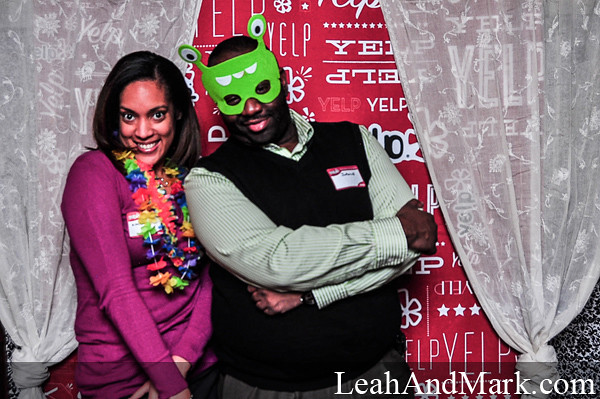In this vivid, colorful image, a woman and a man are posing together in front of a red Yelp step-and-repeat banner, flanked by white curtains. The woman, standing on the left, has long brunette hair and large, expressive eyes as she smiles at the camera. She is adorned with a vibrant paper lei around her neck and wears a long-sleeved fuchsia magenta sweater. A name badge is visible on her attire. Beside her stands a man, an approximate age between 35 and 40 years, wearing a green mask that covers the top half of his face in the depiction of a cartoon character. He is dressed in a long-sleeved green shirt under a black vest, and his arms are folded across his midsection. Both individuals have name tags. The photo is bright and clear, capturing the lively and festive atmosphere of the event. In the bottom right corner of the image, the text "Leia and Mark dot com" is visible, adding an additional detail to the scene.